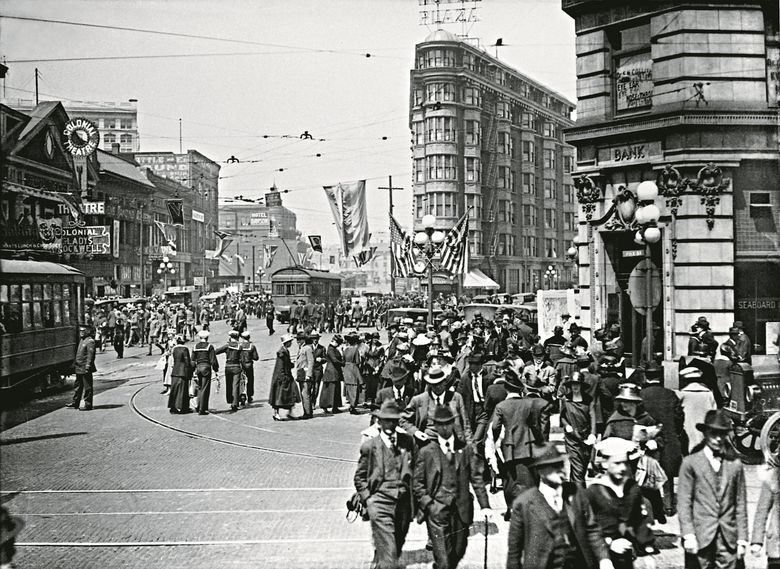This black and white photo, likely from the 1920s, captures a bustling street scene at a three-way intersection. The image is filled with people, many of whom are dressed in suits and hats, while a few sailors are also visible. Women are elegantly attired in long gowns, coats, and hats, suggesting they are dressed for a special event. The street is crowded with pedestrians, carriages, bicycles, and trolley cars, which run on tracks embedded in the brick-paved streets, creating a lively urban atmosphere.

On the right side of the image, a prominent bank building stands on the corner, its signage clearly indicating its purpose. On the left side, a colonial-style theater with a sign reading "Golden Mill Theater" adds to the historical ambiance. American flags are displayed in various parts of the scene, with one flag prominently hanging down into the cityscape.

Cable car wires are strung between the buildings, contributing to the image's classic city feel, possibly reminiscent of San Francisco. The overall scene is vibrant and lively, saturated with the movement and interactions of people, and evokes a sense of a community gathering or a special event.